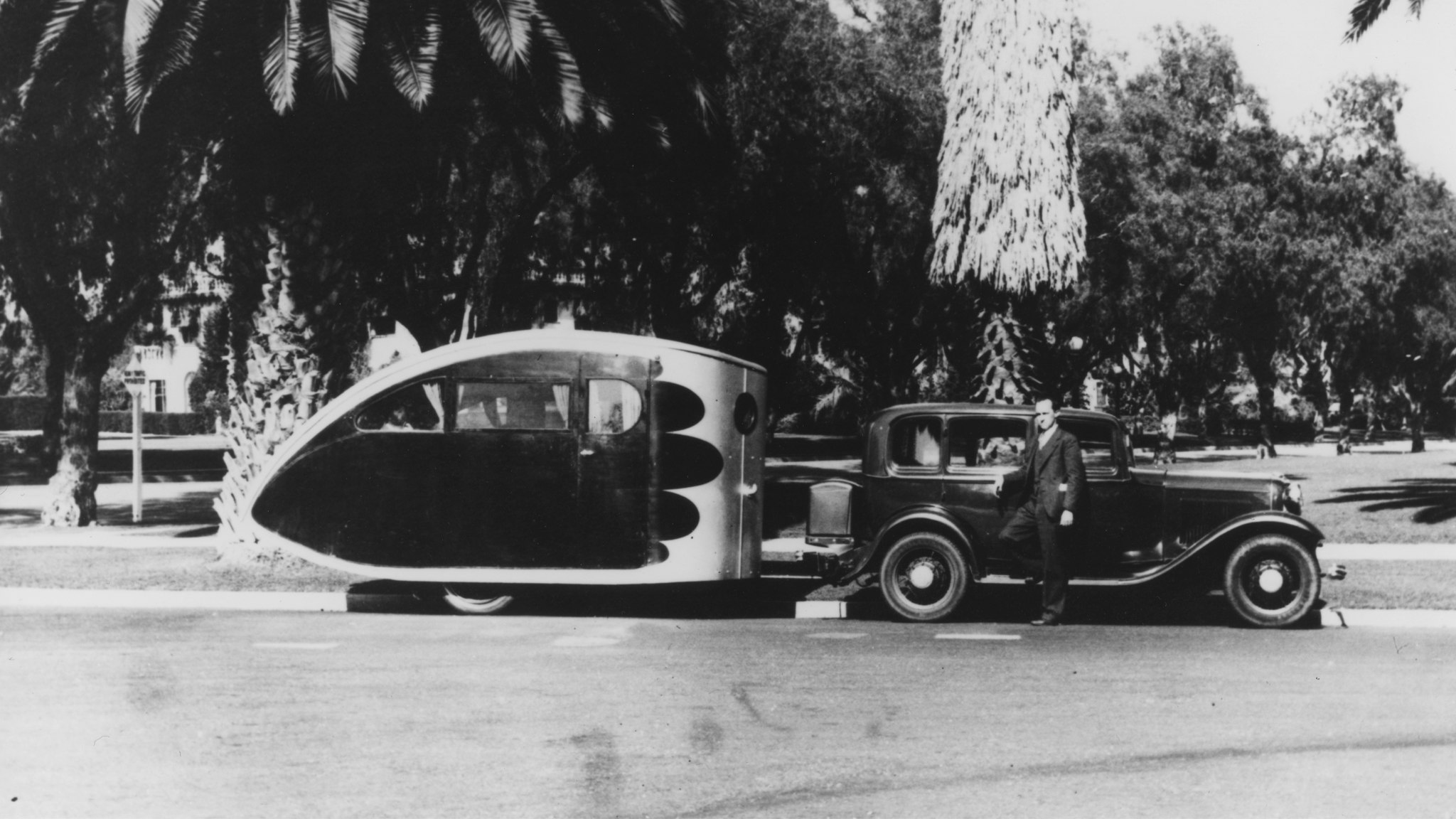This black and white, vintage-style photograph captures an old Model T car parked in a landscape setting, facing to the right of the image. The car is pulling a silver, bullet-shaped trailer with a distinctive black wing design painted on its side. The trailer has a flat front, a curved top, and a slightly upturned bottom, resembling a tail; it also features a door with a silver handle and a couple of windows.

A man dressed in a black suit leans against the car, with his shoulder resting on its glass window and his foot on the car’s step. The car itself has a wide bumper, two wheels, a door, and windows, along with a luggage carrier positioned at the back, right above the trailer hitch.

In the background, there's a variety of trees, prominently including several palm trees, all of which cast shade, given the daytime setting. To the left of the image, a wooden fence with thin posts and two slats is partially visible. The foreground features a gray street, and the sky appears muted, contributing to the photograph's classic, shaded ambiance.